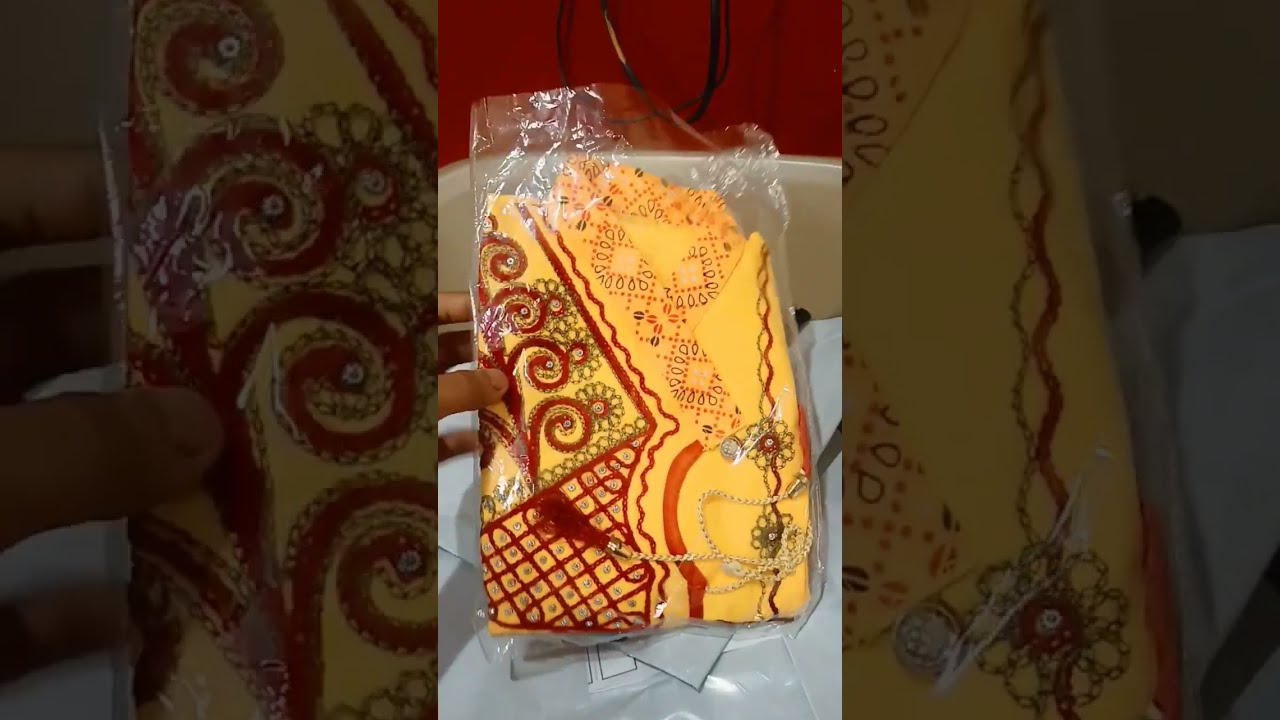The central image, a vibrant color photograph in portrait orientation, features a richly detailed garment inside a clear plastic bag. The garment, primarily a bright mustard yellow with intricate red patterns, is reminiscent of Indian motifs. A prominent detail is the silver cord with a red tassel that accompanies the garment. This plastic package is being held up by a hand entering from the left side of the frame, the fingers of which are brown in color. Behind the plastic package, one can see a brown wooden chair with some white objects beneath it. The backdrop is a distinct red wall intersected by what appears to be a black and white cord. On either side of the central image, the same photograph is enlarged, displayed in landscape orientation, and appears darker and out of focus. The composition is detailed and rich with color, bringing emphasis to the vibrant fabric and its ornate design.